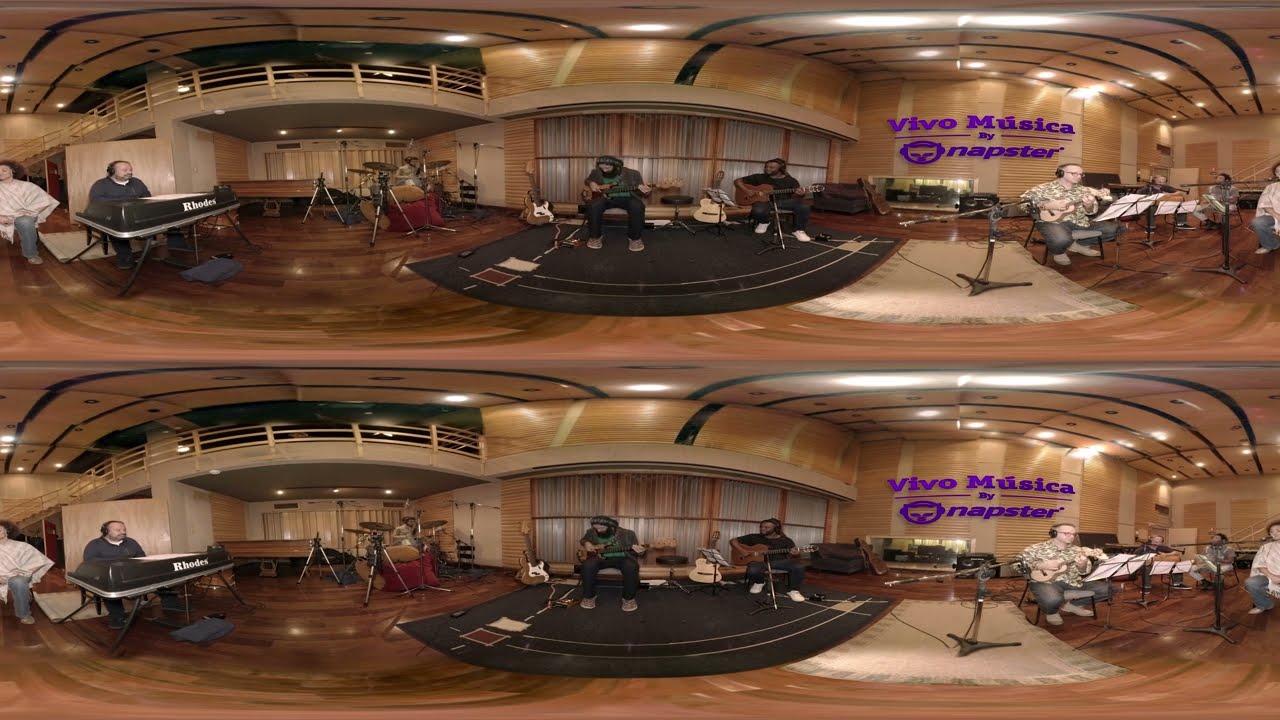The image is a panoramic photograph, composed of three distinct yet seamlessly integrated shots, capturing the dynamic essence of a music session inside a recording studio. The fisheye lens effect creates a captivating, swirly, fishbowl perspective. Central to the scene is the purple text on a wall panel, reading "Vivo Musica by Napster," signifying that the session is sponsored by Napster. 

In the middle section, two men are the focal point, each engrossed in playing a guitar—one with an acoustic guitar and the other with a bass electric guitar. The right section of the image features a man seated with a music folder stand, seemingly holding a mandolin while another individual sits beside him, potentially singing into a microphone. The left section reveals a man seated at a keyboard, with a backdrop of another musician energetically playing the drums. 

The entire setting is enriched with hardwood floors and wood-paneled walls, conveying the warm, authentic ambiance of the studio. A notable architectural feature is the balcony visible in the upper part of the left section. The overall scene vibrantly illustrates a multifaceted music practice or recording session, bustling with creativity and collaborative energy.